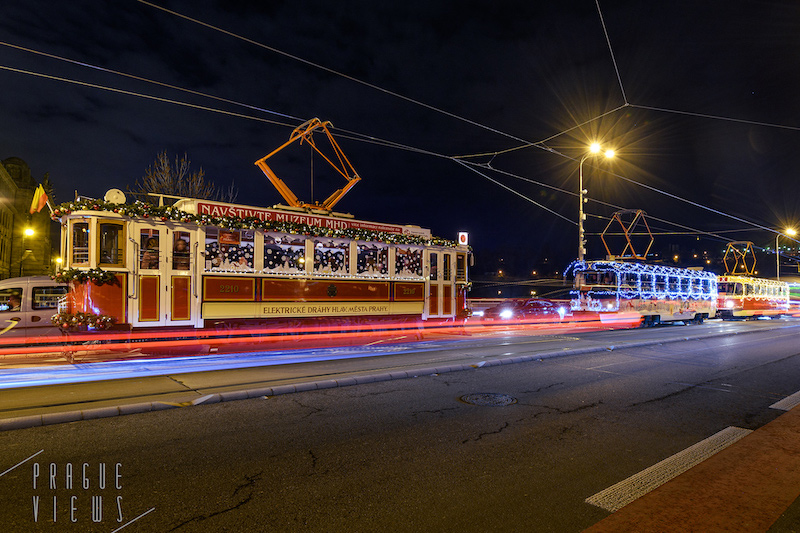This color photograph, taken at night, vividly captures a festive scene featuring three trolley cars on a rail, decorated with greenery and illuminated Christmas lights. The black night sky enhances the brilliance of the illuminated trolleys. Positioned on a highway, the rail track is lit up with intricate red and blue neon lights, creating a striking visual contrast against the dark pavement and clearly marked white road lines.

In the foreground, dark cement pavement and lighter-colored berms bisect the roadway, further accentuated by white lane markings. The main subjects of the image, three trolleys, are attached to overhead electric cables typical of cable cars.

The front trolley is adorned with vibrant greenery and colorful Christmas lights, making it the most visually striking. It bears foreign text, "NAVSTIVTE MUZEUM MHD" and "ELEKTRICKÉ DRÁHY HLAVNÍHO MĚSTA PRAHY," with the number "2210" also visible. The middle trolley is bathed in blue lights, while the rearmost trolley glows with lighter, possibly white or soft blue lights. Additionally, the foreground and the trolley lights create a festive and inviting atmosphere, further signified by the "Prague News" emblem in the bottom left-hand corner, suggesting the location could be Prague.